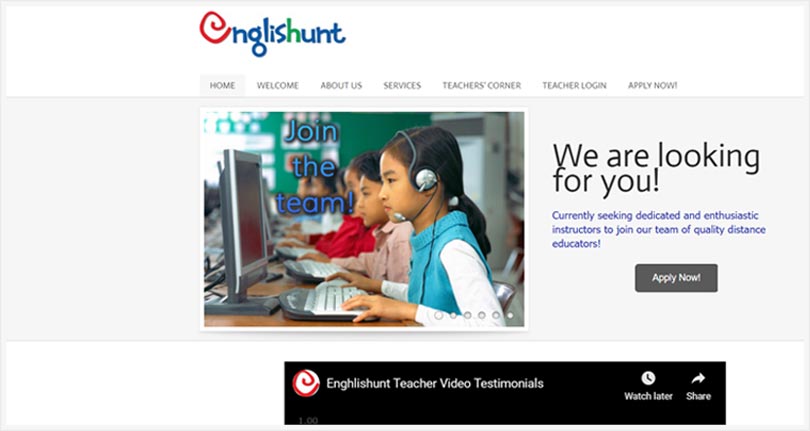This screenshot from a web page showcases the online platform "English Hunt" with its logo prominently displayed at the top in a blend of red, blue, and green. Below the logo, there are several navigation tabs: Home, Welcome, About Us, Services, Teacher's Corner, Teacher Login, and Apply Now. The Home tab is currently selected.

The central portion of the screenshot features a large image depicting a row of students engrossed in their work on computers, each wearing silver headphones that match their silver monitors and keyboards. In the foreground, a girl wearing a white long-sleeve shirt paired with a turquoise vest concentrates on her screen. Beside her, a young man in a light pink button-up shirt works diligently, followed by another student in a red shirt.

To the right of the photograph, a welcoming message reads: "We are looking for you," followed by blue text that invites passionate educators to join the platform: "Currently seeking dedicated and enthusiastic instructors to join our team of quality distance educators. Apply now."

At the bottom of the screen, a black bar displays the prompt "English Hunt teacher video testimonial," accompanied by options to "Watch later or save." This section likely offers insight from current educators about their experiences with the platform.